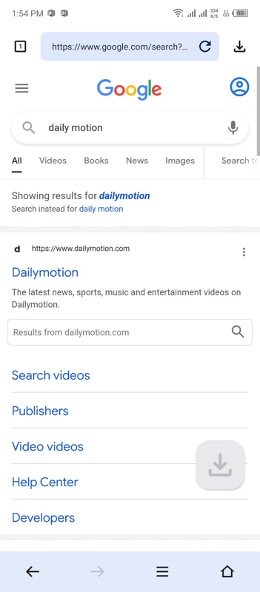In this screenshot taken from a phone, the Google search interface is prominently displayed. The iconic Google logo is shown in its rainbow-colored font at the top. Above the logo, there is the URL of a webpage, and at the very top left corner, the time reads 1:54 PM. To the right of the time, multiple icons indicate the phone's Wi-Fi connection, battery usage, and other status indicators.

The search box below the Google logo features an arrow curved downwards to the lower right, pointing towards a download icon. Within the search bar, "Dailymotion" is typed out, accompanied by a magnifying glass icon on the left side and a microphone icon on the right. Next to the Google logo, a profile icon is also visible.

Underneath the search bar, the term "Dailymotion" is repeated in a smaller format, followed by options categorized as All, Videos, Books, News, and Images. It states, "Showing results for Dailymotion," with "Dailymotion" highlighted in blue, while the rest of the text is in gray. Below this, there's an option in lighter blue text that reads "Search instead for Dailymotion."

A gray separator line follows, leading to the first search result which contains the Dailymotion URL along with a bold "D" icon on the left and three descriptive lines next to it. The result in blue reads, "Dailymotion - Explore the latest news, sports, music, and entertainment videos on Dailymotion."

Further down, additional search results from Dailymotion.com are listed, including options such as Search Videos, Publishers, Video Videos, Help Center, and Developers. A download button is positioned between "Video Videos" and "Help Center" on the right. Another gray line separates this section from the navigation bar at the bottom of the screen.

The navigation bar features icons including a dark arrow pointing left, a lighter arrow pointing right, a three-line menu icon, and a house icon on the lower right-hand side.